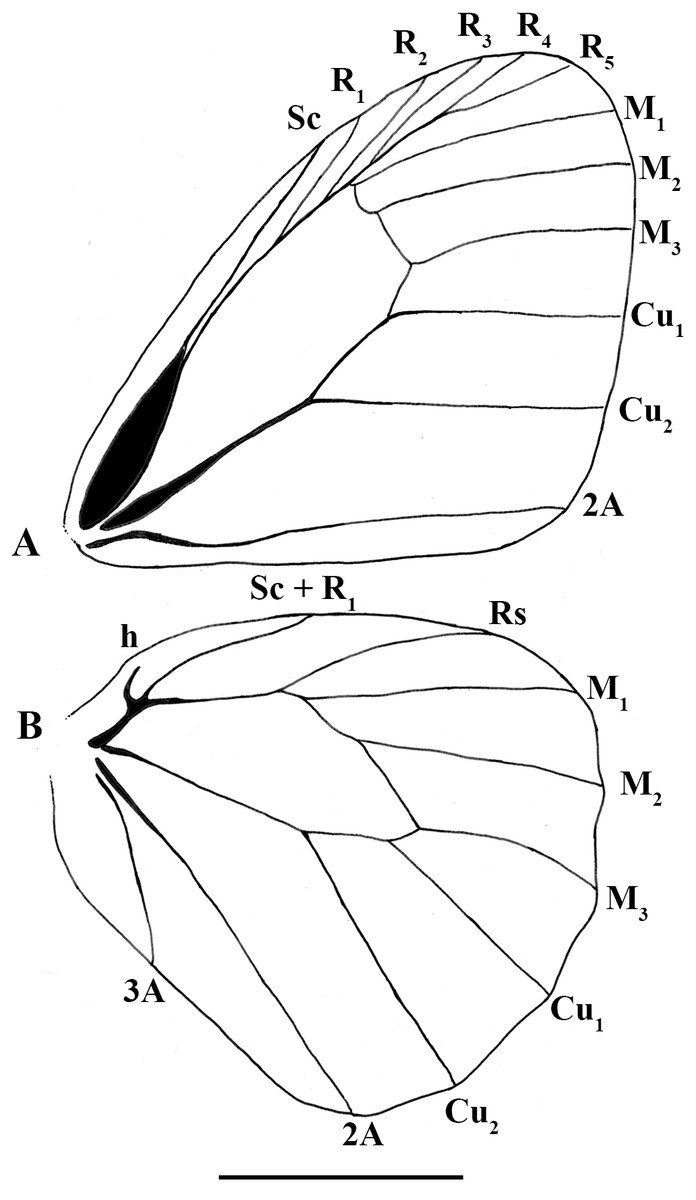The image is a detailed black and white diagram featuring two distinct structures labeled A and B. Both structures resemble insect wings, specifically those of a butterfly, though B also somewhat resembles a leaf. Structure A, situated on top, is meticulously marked with various lines and sections that denote anatomical features. These sections are labeled with a combination of letters and numbers, including SC, R1 through R5, and CU1 and CU2, M1 through M3, and 2A at the bottom. Structure B, located below A, has a similar labeling system with SC, RS, M1 through M3, CU1 and CU2, and 2A. Both wings exhibit intricate vein-like patterns that delineate the different segments, suggesting a focus on the morphology and structure of butterfly wings.